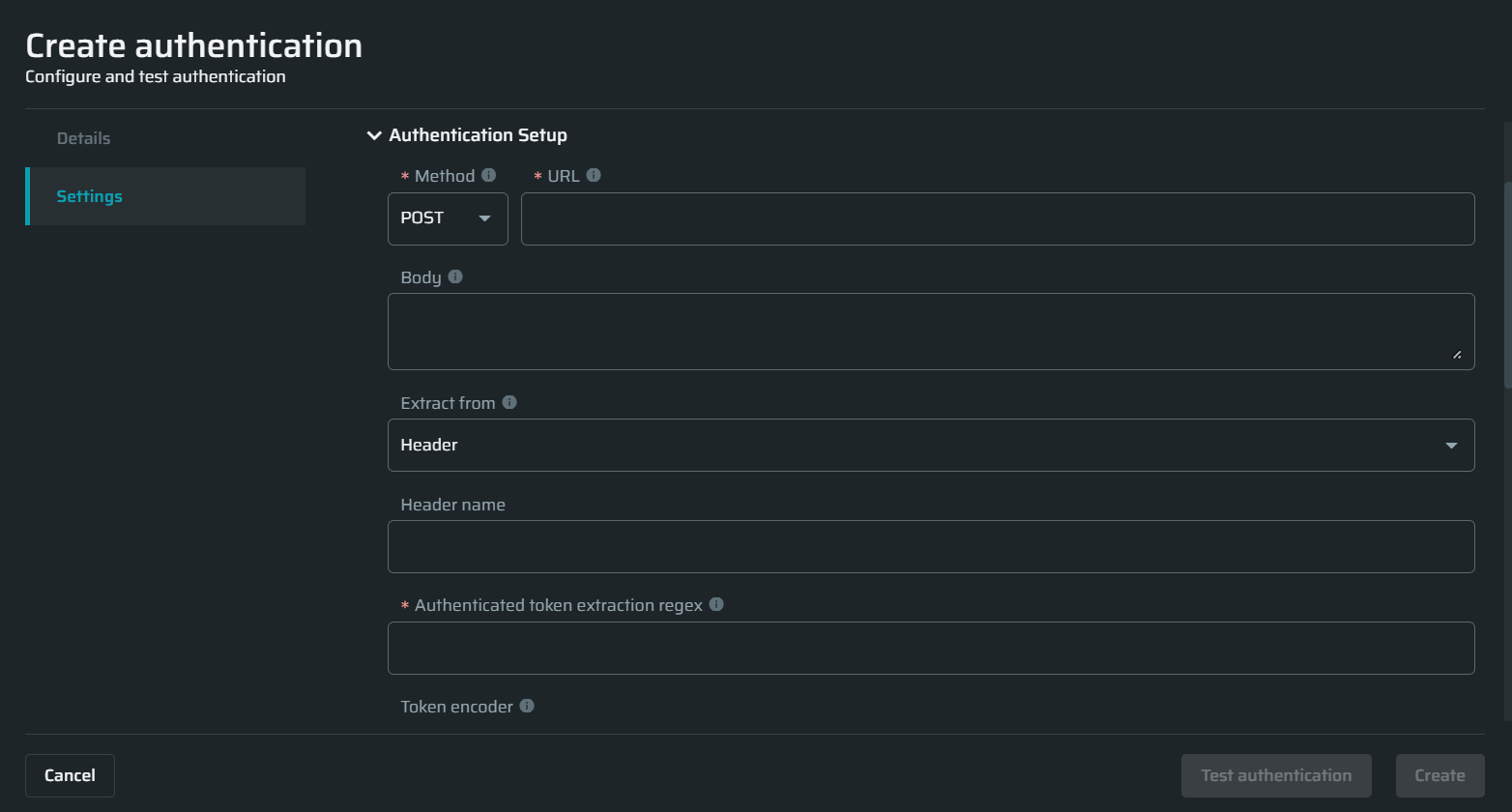The screenshot displays a user interface on a black background with white text, specifically from a web authentication configuration page. 

In the top left corner, the heading "Create Authentication" is prominently displayed. Directly below it, the subheading reads "Configure and Test Authentication." A faint horizontal line separates this section from the content beneath.

On the left side, the section titled "Details" is visible, accompanied by a lighter-colored box labeled "Settings" highlighted in blue. To the right of this box, there is an arrow indicating a dropdown menu for additional settings options.

The interface contains several input fields for configuring the authentication setup. The first input field labeled "Method" has a preset value of "POST" and includes a dropdown menu for selecting different HTTP methods. The subsequent field is a long text box designed for entering a URL.

Below the URL field, there is a "Body" section featuring a large text area intended for inputting the request body data. Following this, the "Extract From" section contains a text box with the word "header" pre-filled, indicating where to extract key information from the response.

Subsequently, there is an empty text box labeled "Header Name" for specifying the header from which to extract data. Another empty box titled "Authenticated Token Extraction REGX" is provided, presumably for entering regular expressions to extract authentication tokens.

The final option, "Token Encoder," appears below the token extraction field. At the bottom right of the interface, there are two prominent buttons: "Test Authentication" and "Create," offering options to test the configuration or create the authentication settings respectively.